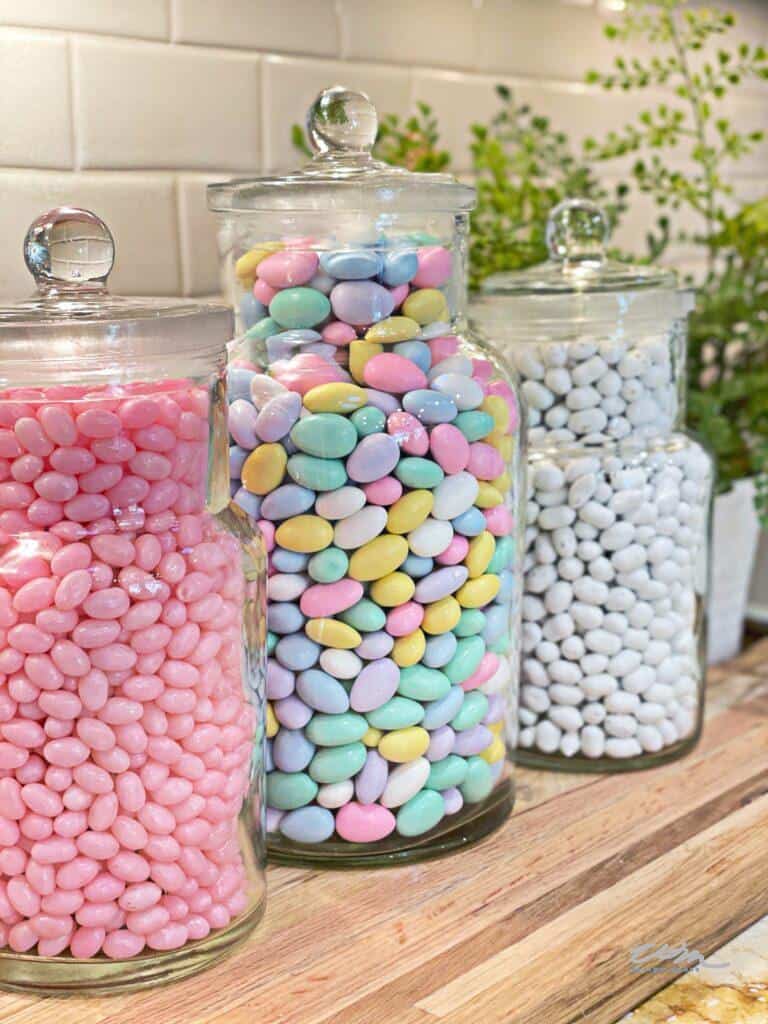This photograph captures a neatly arranged trio of clear glass candy jars set against a white subway tile backsplash with horizontal patterns in a kitchen setting. The jars, each topped with a glass knob lid, sit on a wooden countertop. The jar on the left contains pink jelly beans, while the taller central jar is filled with pastel-colored Jordan almonds—in hues of purple, green, white, yellow, and pink. The jar on the right houses white candy, possibly white raisinets or white jelly beans. In the background, a slightly blurred green plant adds a touch of natural decor. Subtle, hard-to-read, silver squiggles at the bottom of the image might indicate a name or signature.